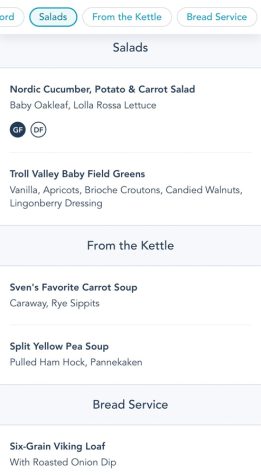The image is a vertically rectangular cell phone screenshot, likely taken from a restaurant's digital menu. The interface shows a series of buttons aligned horizontally at the top, highlighted with the current section titled "Salads." Beneath this, the screen is divided into three main sections, each with a heading. 

The first section, marked by the heading "Salads" in a light gray banner, lists the following items on a white background:
- Nordic Cucumber, Potato, and Carrot Salad
- Baby Oak Leaf and Lola Rosa Lettuce
- Troll Valley Baby Field Greens
- Vanilla Apricots
- Brioche Croutons
- Candied Walnuts
- Lingonberry Dressing

The second section features "From the Kettle," also highlighted by a light gray banner, with the following items on a white background:
- Sven's Favorite Carrot Soup
- Carraway Rye Sippets
- Split Yellow Pea Soup
- Pulled Ham Hock
- Penne Cacken

The third and final section is titled "Bread Service," again on a light gray banner, listing:
- Six Grain Viking Loaf with Roasted Onion Dip

Each heading is distinctly marked on a light gray banner, while the individual menu items are presented on a white background, ensuring clear readability and organization.